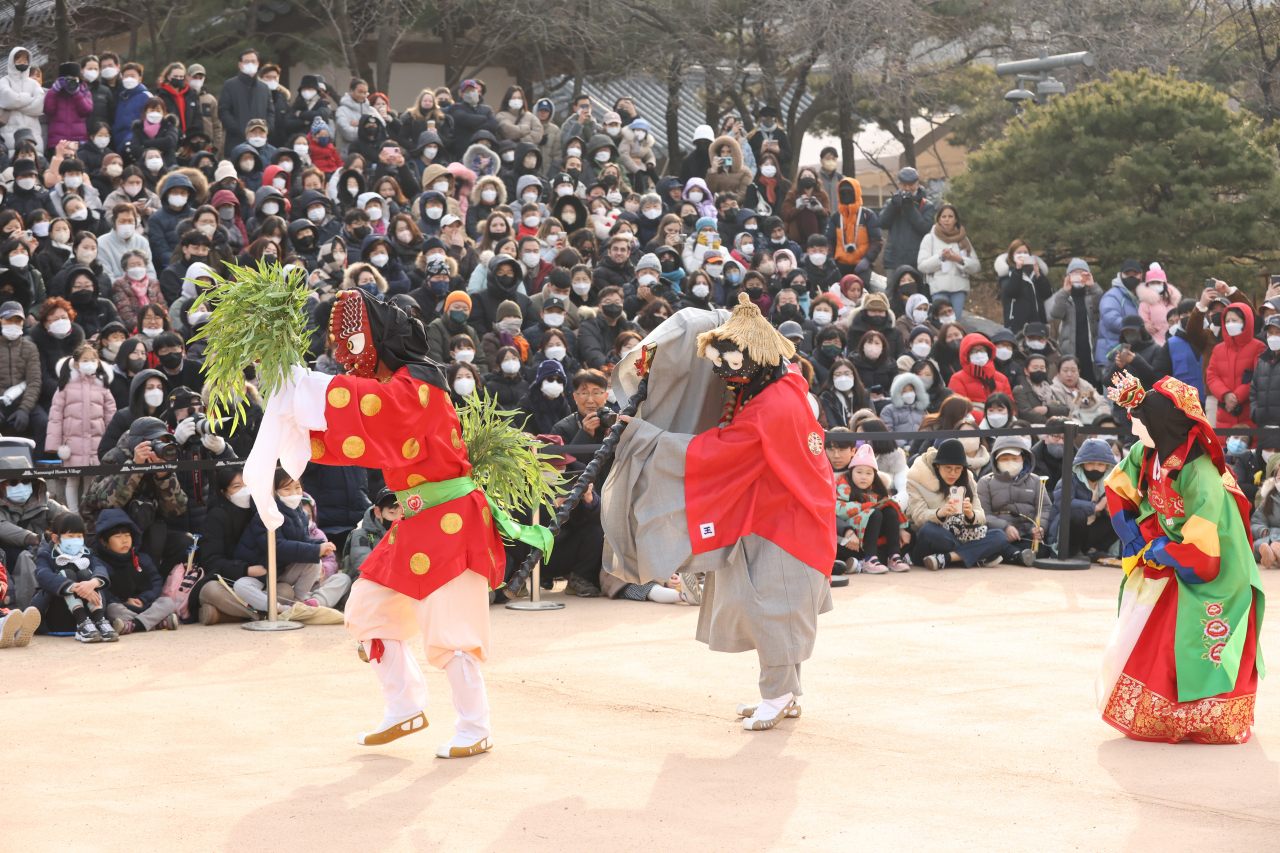This detailed photograph captures a lively outdoor performance set on a flat stage, surrounded by a diverse audience. The scene takes place during the day, with trees and buildings dotting the background. On a small hill in the distance, spectators are seated, fully engaged and capturing the moment with cameras. The audience is adorned in a variety of colorful jackets—black, pink, white, gray, red, blue, beige, and patterned—and everyone is wearing masks, indicative of COVID-19 precautions.

The focal point of the image is three performers positioned from left to right center. They are dressed in traditional, vividly colored costumes, bringing a folkloric scene to life. The leftmost performer, seemingly dancing, dons a red mask with a single white eye and a yellow pupil. They are dressed in a kimono with orange-yellow dots, a light green waist band, white pants, socks, and light brown sandals, and they hold branches with large leaves in both hands.

The middle performer wears a beige kimono with a red shirt over it, paired with light brown sandals and white socks. They also feature a weaved light brown cap and a straw hat, along with a black mask designed to resemble a monstrous face.

The performer on the right embodies intricate vibrancy, garbed in a red kimono with an elaborate light green kimono over it, the sleeves adorned with yellow, red, and blue hues. They also wear a black hood and a mask with a white face, adding to their mystique.

Overall, the photograph captures a rich tapestry of tradition, performance, and community, vividly displaying both the elaborate costumes of the performers and the captivated, colorful attire of the audience.